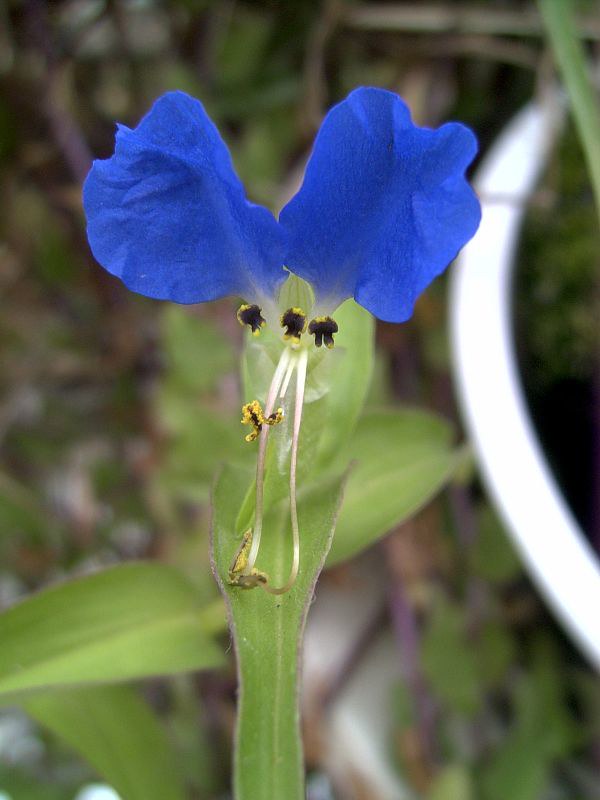This is a photo featuring a striking blue flower with two large, vibrant blue petals. The flower is just beginning to sprout, with intricate details at its center, including yellow and black seeds and delicate white vines. The flower is surrounded by green leaves and appears to be part of a larger batch of flowers. In the background, there are blurred trees, bushes, and some dirt and debris. Notably, there is a glowing white circle to the right of the flower, adding an intriguing element to the image. The darker square around the edge frames this luminous and detailed botanical scene.